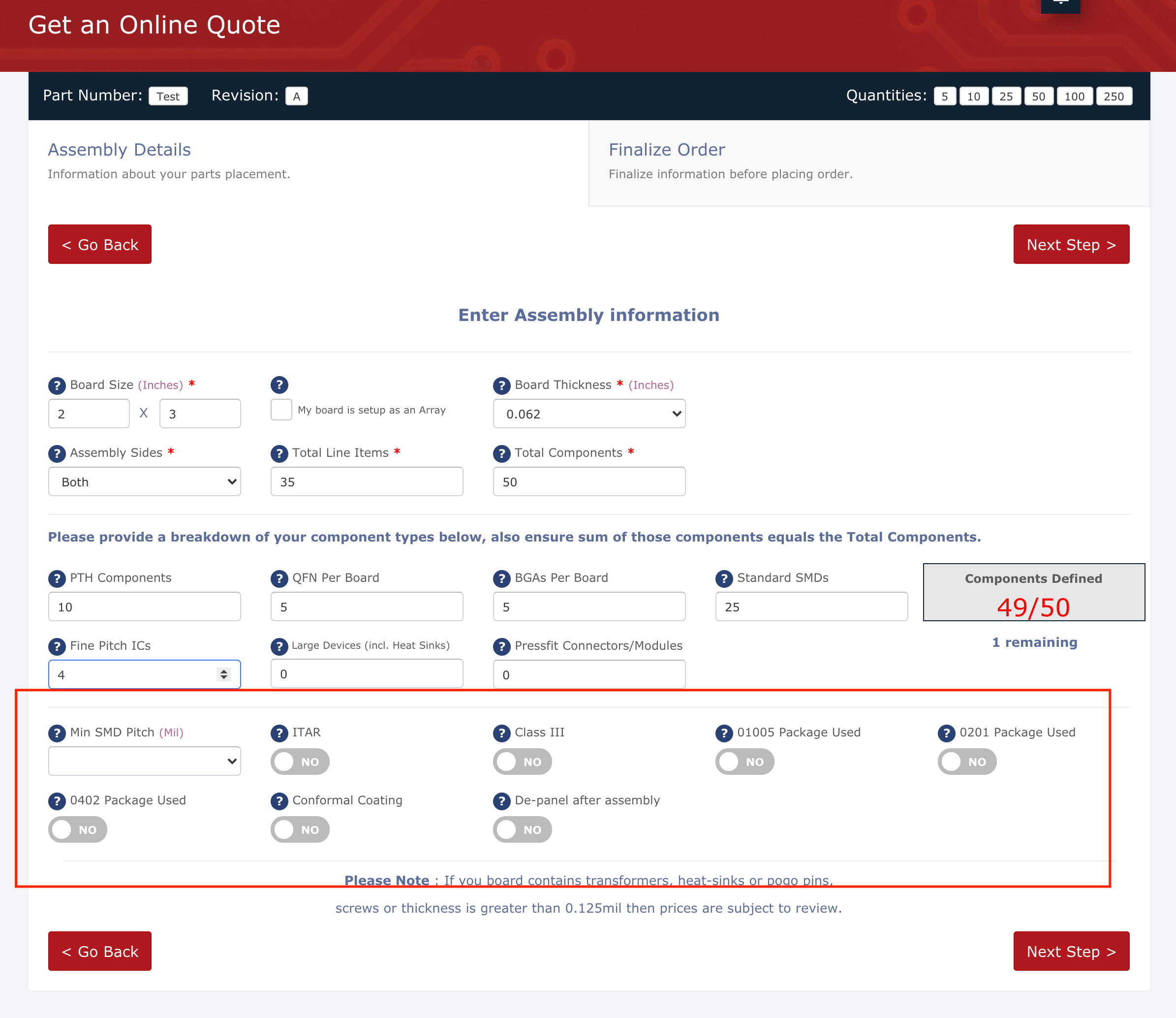This screenshot, taken from a website offering online quotes for services, features a navigation bar at the top left with the text "Get an Online Quote" prominently displayed in white font within a red bar that spans the width of the image.

Below the navigation bar, a section outlined with a thin red line catches the eye. This section contains a text drop-down arrow menu prompting users to select their desired minimum SMD pitch. Subsequent to this menu are columns with checkboxes that seem to be set parameters for customization:

1. The first checkbox, labeled "0402 Package Used," is set to 'No.'
2. The second checkbox, labeled "ITAR," is set to 'No.'
3. The third checkbox, labeled "Conformal Coding," is set to 'No.'
4. The fourth checkbox, labeled "Class 3," is set to 'No.'
5. The fifth checkbox, labeled "Depanel After Assembly," is set to 'No.'
6. The sixth checkbox, labeled "01005 Package Used," is set to 'No.'
7. The seventh and final checkbox, labeled "0201 Package Used," is also set to 'No.'

This structured layout emphasizes the variety of selectable options available for the user to configure according to their specific requirements.